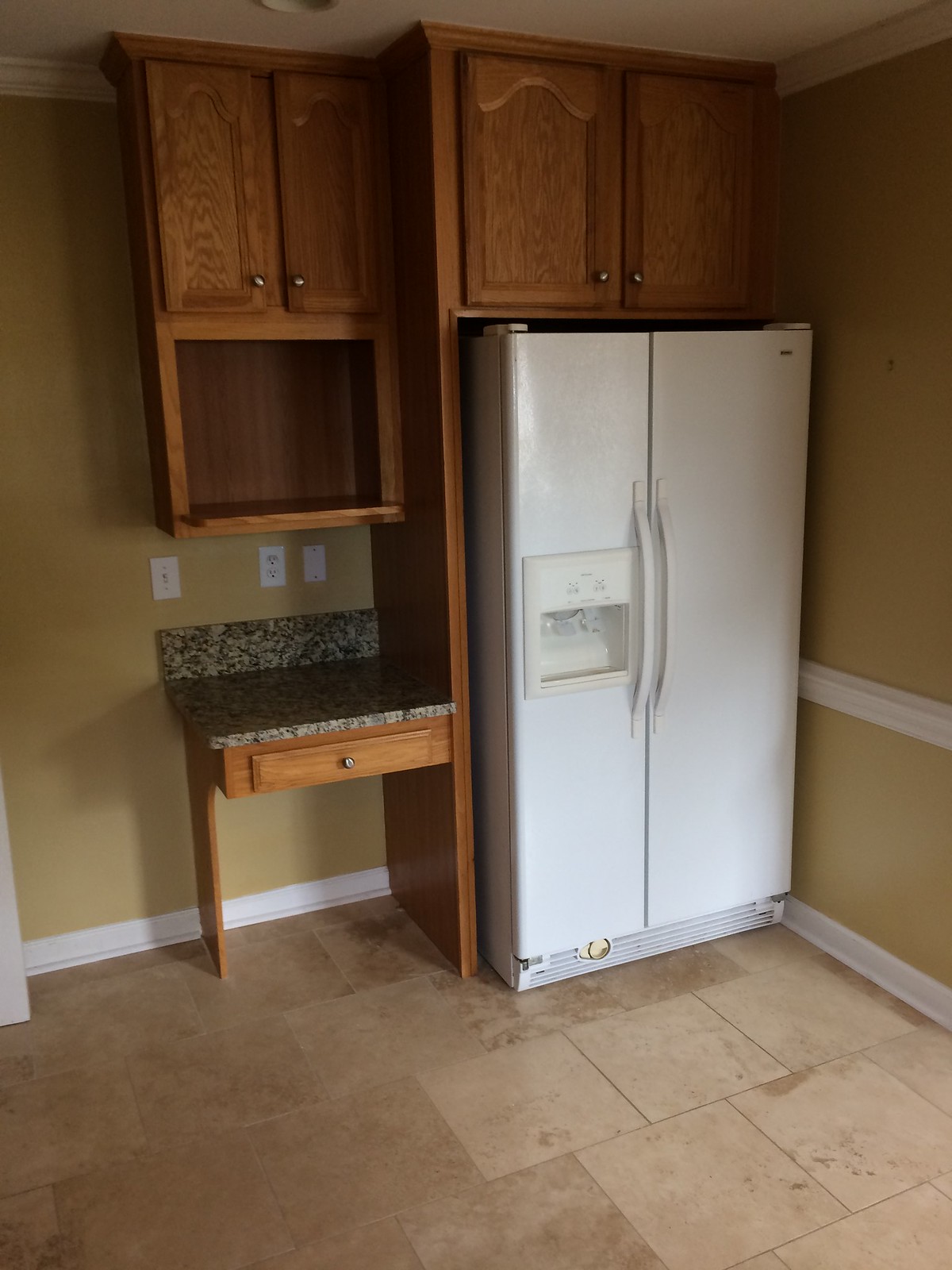The photograph captures an empty kitchen, suggesting a home in the midst of move-in or move-out. The kitchen features a two-door white refrigerator with a built-in ice and water dispenser, snugly fit into an alcove formed by light-colored oak cabinets. Directly above the fridge, there is a dual-door cabinet for additional storage. To the left of the refrigerator is a compact wooden table or desk, also topped with a granite-like surface with a mix of green, brown, tan, and silver hues. The kitchen floor is noticeably tiled in two distinct shades, indicative of a repair that required relaying parts of the floor. The walls are painted a warm golden color, contrasted by white trim and chair rail molding that run along the room. Additional features include several electrical outlets and a visible light switch near the small tabletop area. The overall style of the kitchen hints at a design aesthetic from the 1990s.